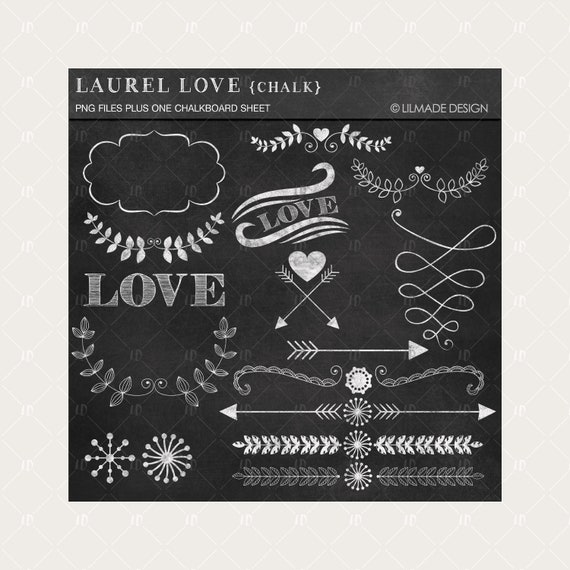The image appears to be a detailed computer graphic that convincingly mimics a real chalk drawing on a dark gray, almost black background. The central feature is a dark gray square with multiple chalk graphic elements in white, varying in boldness. The words "Laurel Love Chalk" are prominently displayed at the top left, accompanied by a notation that reads "PNG files plus one chalkboard sheet". A small copyright symbol on the top right credits "Lil Made Design". Among the intricate designs on the dark gray section, there are several occurrences of the word "love", geometric shapes, crossed arrows with a heart above, squiggly lines, floral wreaths, and other decorative patterns. The overall effect is a rich tapestry of chalk art, showcasing the variety and detail possible with the provided files.